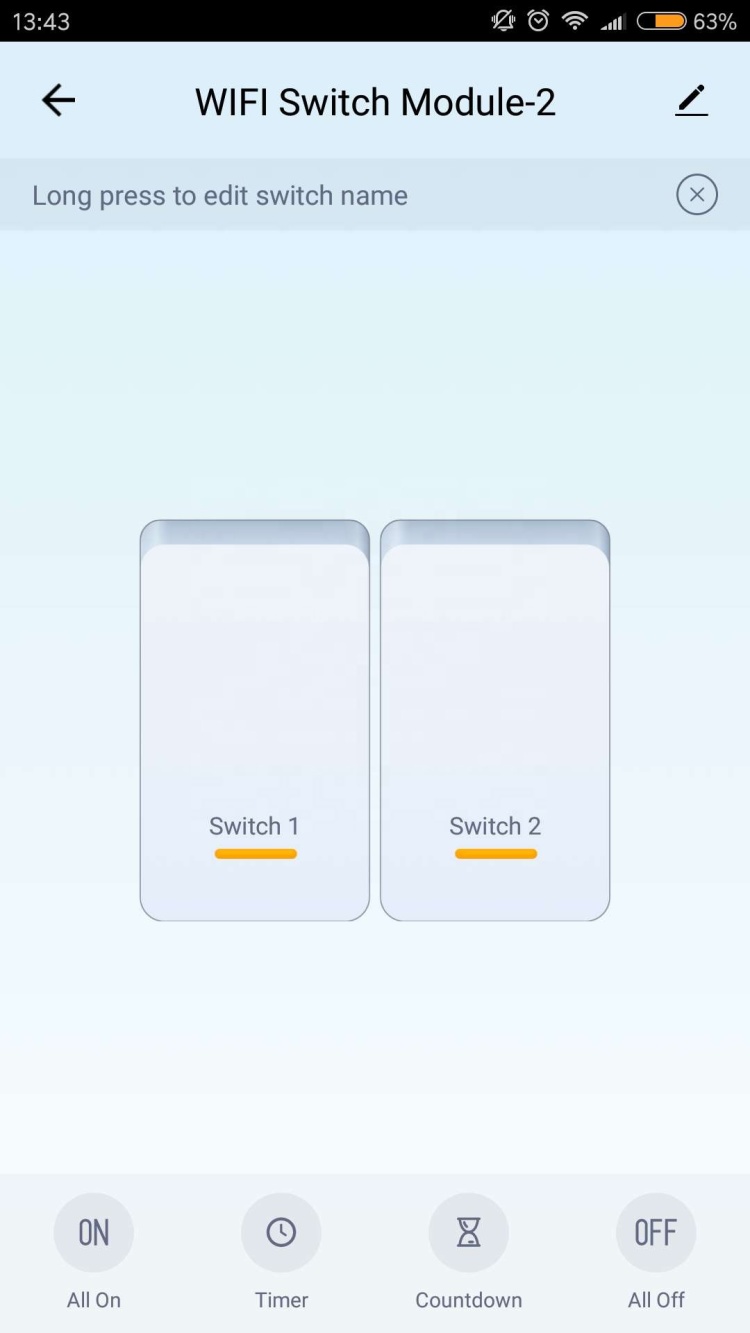The image is a detailed screenshot from an Android mobile app, displaying a control interface for a Wi-Fi switch module. At the top of the screen, a thin black band shows essential system icons, including the time (13:43), an alarm status, connection type and strength, a notification indicator, and battery status both visually and numerically (63% charged). Below this, the heading reads “Wi-Fi switch module-2”, with an arrow icon pointing leftwards adjacent to it, and instructions stating “Long press to edit switch name”.

Central to the screen are two rectangular, smooth-cornered buttons labelled “Switch 1” on the left and “Switch 2” on the right. These are set against a light blue background. At the bottom of the display, a black band houses four options: “All On”, “Timer”, “Countdown”, and “All Off”. The predominant colors in the screenshot are black, white, orange, light blue, and gray. The layout clearly delineates the functional areas with the heading and edit prompts at the top, the switches centrally positioned, and the control buttons lined up at the bottom.